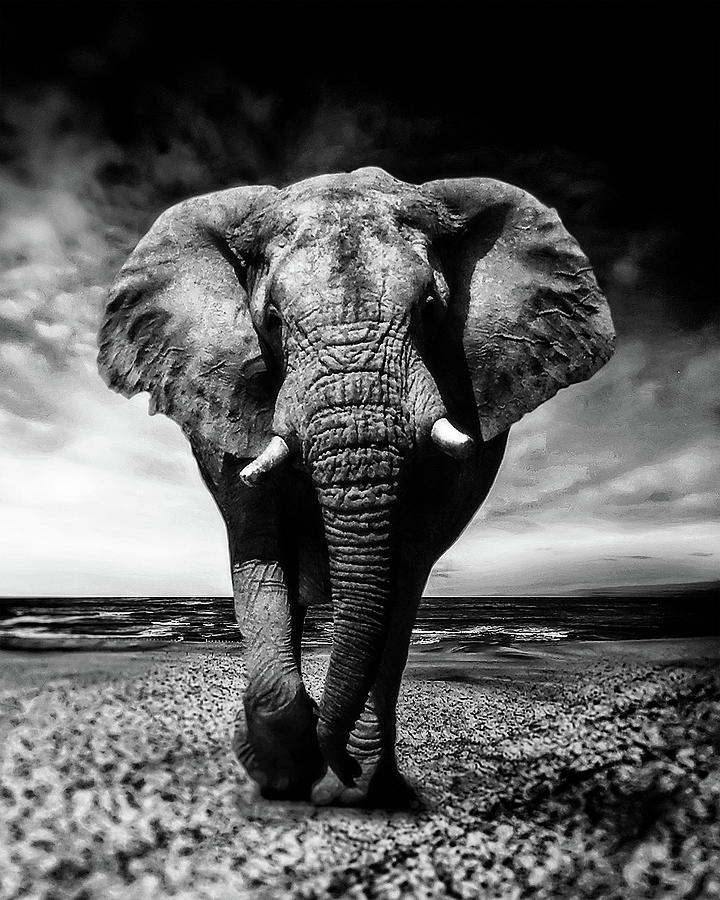In this black-and-white photograph, an African elephant dominates the scene, captured in a frontal view as it appears to be walking towards the camera. The elephant, with its rough, dry skin, slightly bent right leg, and snout hanging down, stands powerfully on the dry, parched land. Its large, prominent ears flank its head, partially shadowing its eyes. Small white tusks protrude from underneath its trunk. The sky overhead is a striking gradient from dark black clouds at the top to lighter gray and near white at the horizon, filled with an array of cloudy textures. Behind the elephant, the horizon blurs with a patchy, dark surface which might be ripples of water or simply the continuation of the rugged terrain. The foreground's bottom corners are slightly blurry, giving the image a soft edge. The detailed, rough ground contrasts sharply with the dark, textured sky, creating a dramatic and awe-inspiring scene.